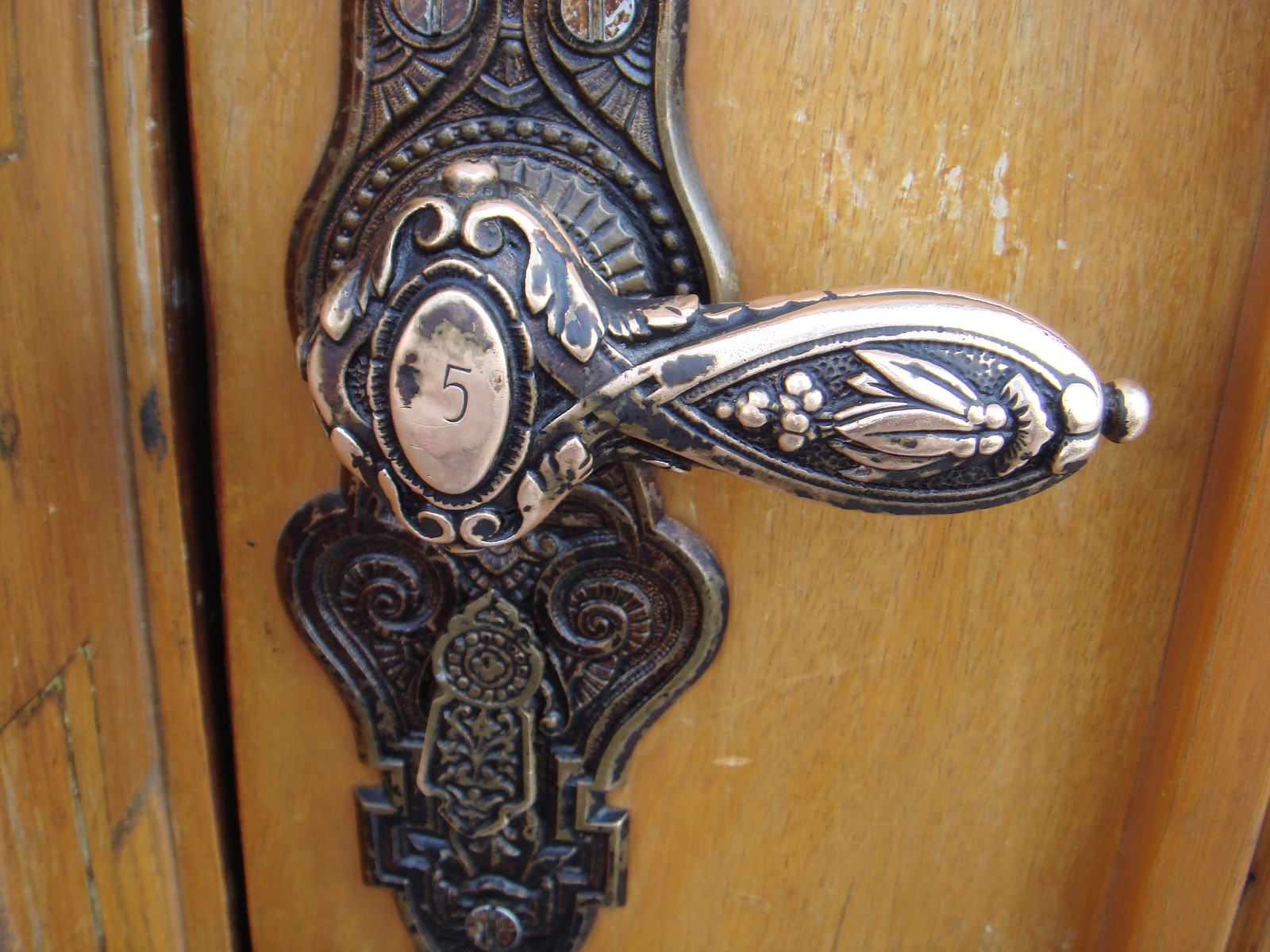This close-up photograph captures an intricately designed, aged door handle on a worn wooden door. The handle, made of metal, predominantly black, reveals patches of worn-off black, exposing a brass or coppery undertone. The handle is a short, thick piece that extends horizontally towards the right-hand side of the image and is designed to function more like a lever. Above the handle is a vertically oriented oval plate featuring an engraved number five and adorned with ornate floral and leaf-like filigree detailing. The door, a light to medium oak wood color, exhibits numerous scratches, blemishes, and faded areas, indicating its age and wear. The background extends to the left, showing a wall of the same material as the door, maintaining a harmonious, yet weathered, appearance.